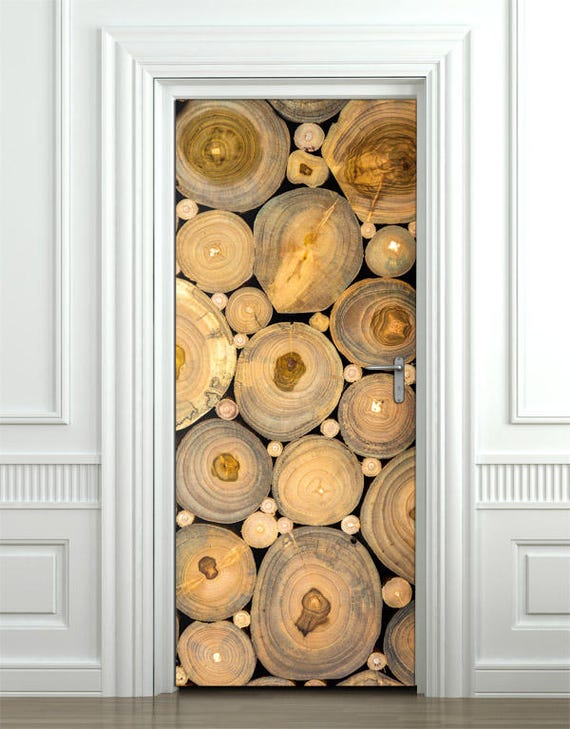The image showcases a creative and innovative door, framed by ornate, colonial-style crown molding and half baseboards along white, textured-pattern walls. The door itself features a metallic silver lever handle and a striking graphic that emulates a stack of sawed-off logs and branches, with visible growth rings illustrating the age of each log. The logs on the door sticker vary in size, with smaller logs interspersed among larger ones, creating a visually intriguing pattern. Complementing this distinctive door, the floor is a reflective, light brown wooden surface, adding warmth to the scene. The door's design is both unconventional and artistic, capturing attention with its unique, detailed depiction of cross-sectional log cuts.